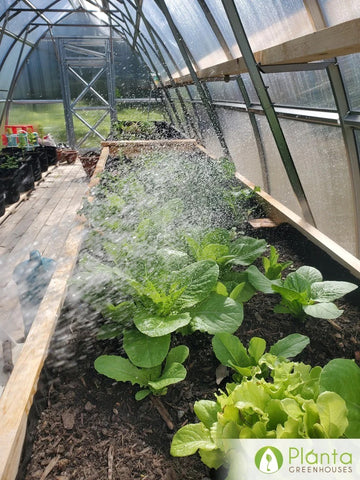The image depicts a verdant scene inside a greenhouse, with a structure characterized by an arched form that tapers to a point at the center above the door at the far end. The greenhouse, constructed from aluminum metal framing, is covered with a slightly foggy, plastic-like material that allows sunlight to filter through, illuminating the plants within. Inside, wooden-raised flower beds or shelves line the walkway, filled with rich brown soil from which various green plants and vegetables, potentially lettuce among them, emerge with different kinds of leaves.

Water droplets can be seen in the air, indicating that the plants are being watered, creating a refreshing spray that adds a dynamic texture to the image. The clear sunny day outside allows plenty of sunlight to penetrate the transparent covering, providing the necessary light for the plants to thrive. Alongside this, there are protective railings and barricades adding structure and order to the scene. At the bottom right corner of the picture, there is a small white rectangle with the text "Planta" in green and "Greenhouses" in a darker brown text underneath. Additionally, a green leaf logo within a circular green border is present, symbolizing the brand, "Planta Greenhouses."